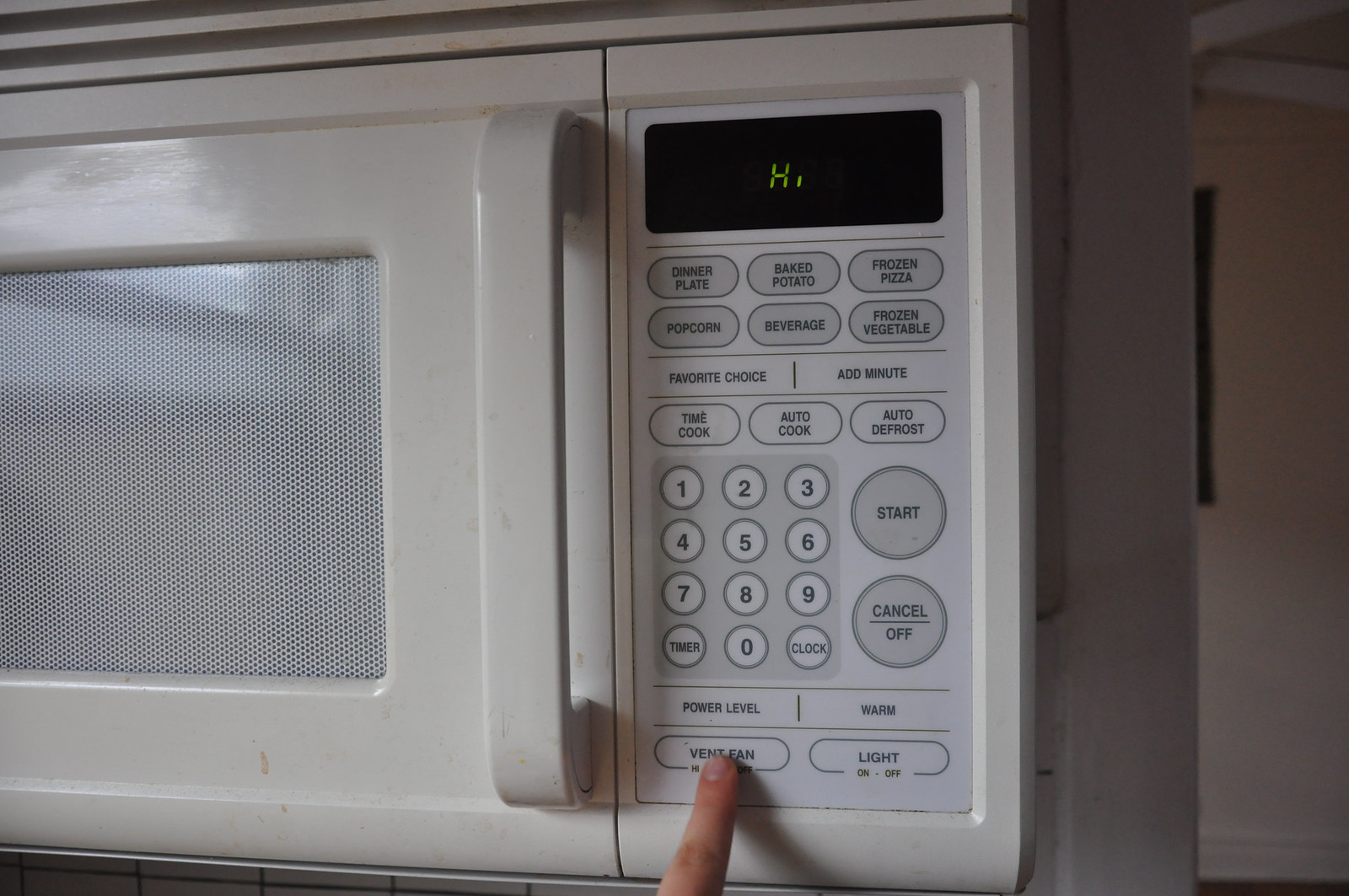This color photograph features a cream-colored microwave oven partially visible from the right-hand side. The microwave door, with a white handle and gray grid-like window, is closed. To the right are various control buttons, encased in a rectangular black panel with "Hi" displayed in lime green on a small screen at the top. Below this screen, numerous buttons offer multiple cooking options, such as baked potato, frozen pizza, beverage, frozen vegetables, dinner plate, and popcorn. Numeric keys from 0 to 9, a start button, and a cancel/off button are also visible.

Centered at the bottom of the frame is a long, skinny finger pressing a button labeled "vent fan." The background reveals a dark gray corridor wall leading to a hallway bathed in light, with a glimpse of a framed picture and gray skirting boards at both the top and bottom of the wall.